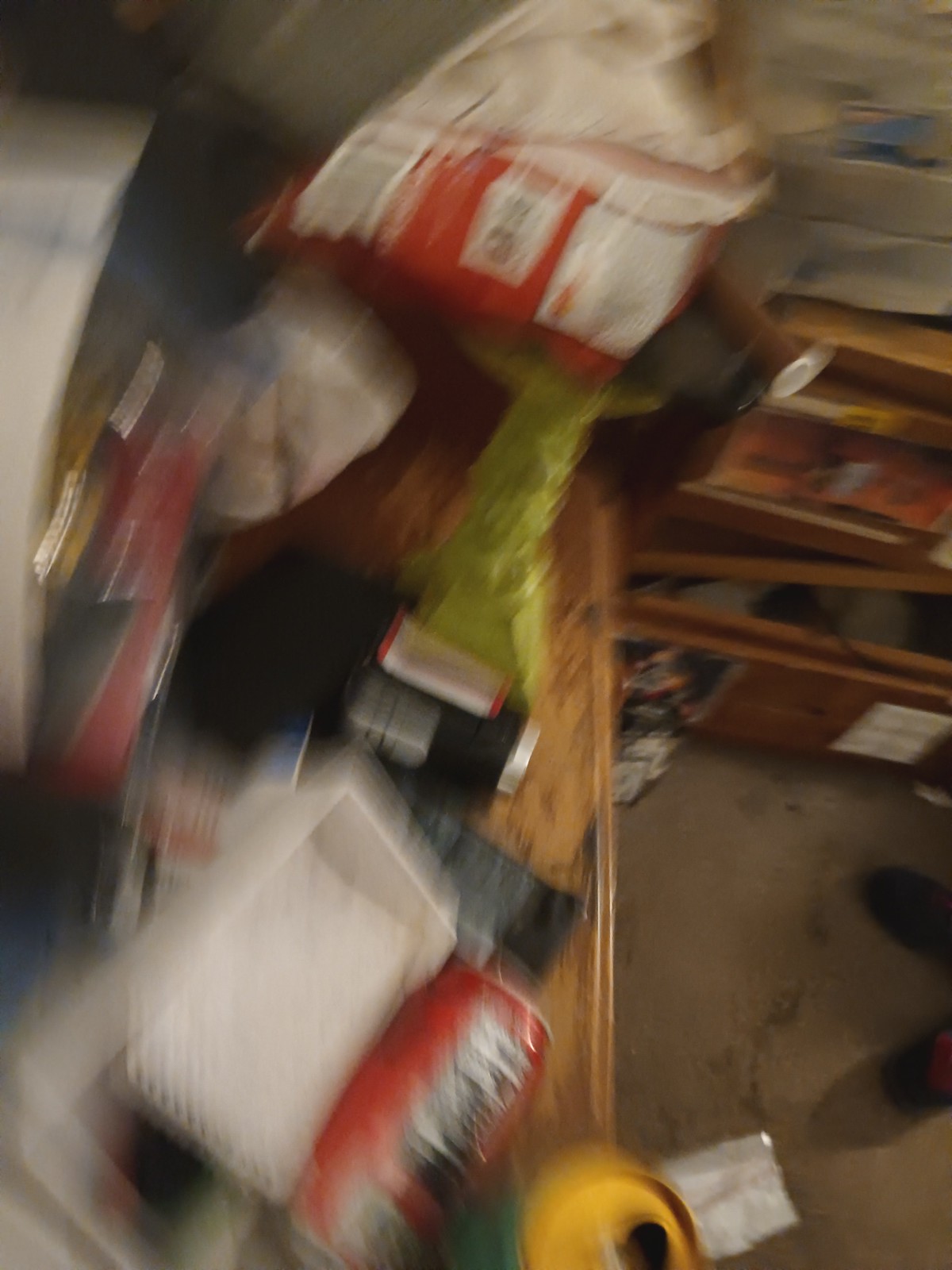In this cluttered storeroom, a mix of disarray and varied items fills the scene. At the center is a very messy desk, prominently featuring a red bag atop it. Nearby, a red can is overturned, while a green can with yellow lids stands upright. Scattered across the desk are a notebook, a lighter, and some kind of foil, adding to the general chaos. To the right side of the image, the concrete floor is marked with oil stains, and wooden shelves flank this area. These shelves are disheveled, with pieces of wood leaning haphazardly against them. The topmost shelf has paper tacked to the wall behind it. At the bottom of the image, partially visible shoes poke out, hinting at either a person or more clutter beneath the desk. A mysterious black object completes the scene, adding to the overall sense of messiness and neglect.